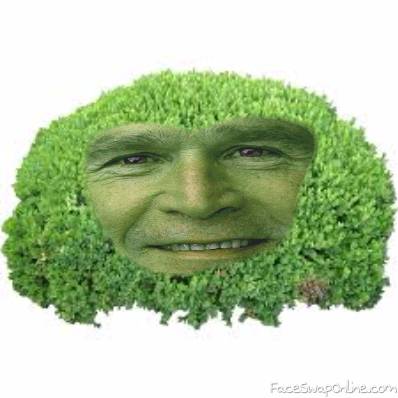The image features a green, plant-like structure reminiscent of a Chia Pet, set against a predominantly white background with a faint light gray square. At its center is a circular pattern of green leaves, and within this greenery is a cutout revealing the photoshopped face of former President George W. Bush. His face is rendered entirely in green hues, with distinct eyes, nose, and mouth, and he is smiling broadly, showing his top row of white teeth and creased eyes. Beneath this central figure, in the lower right-hand corner, is a light gray logo that reads "FaceswapOnline.com".